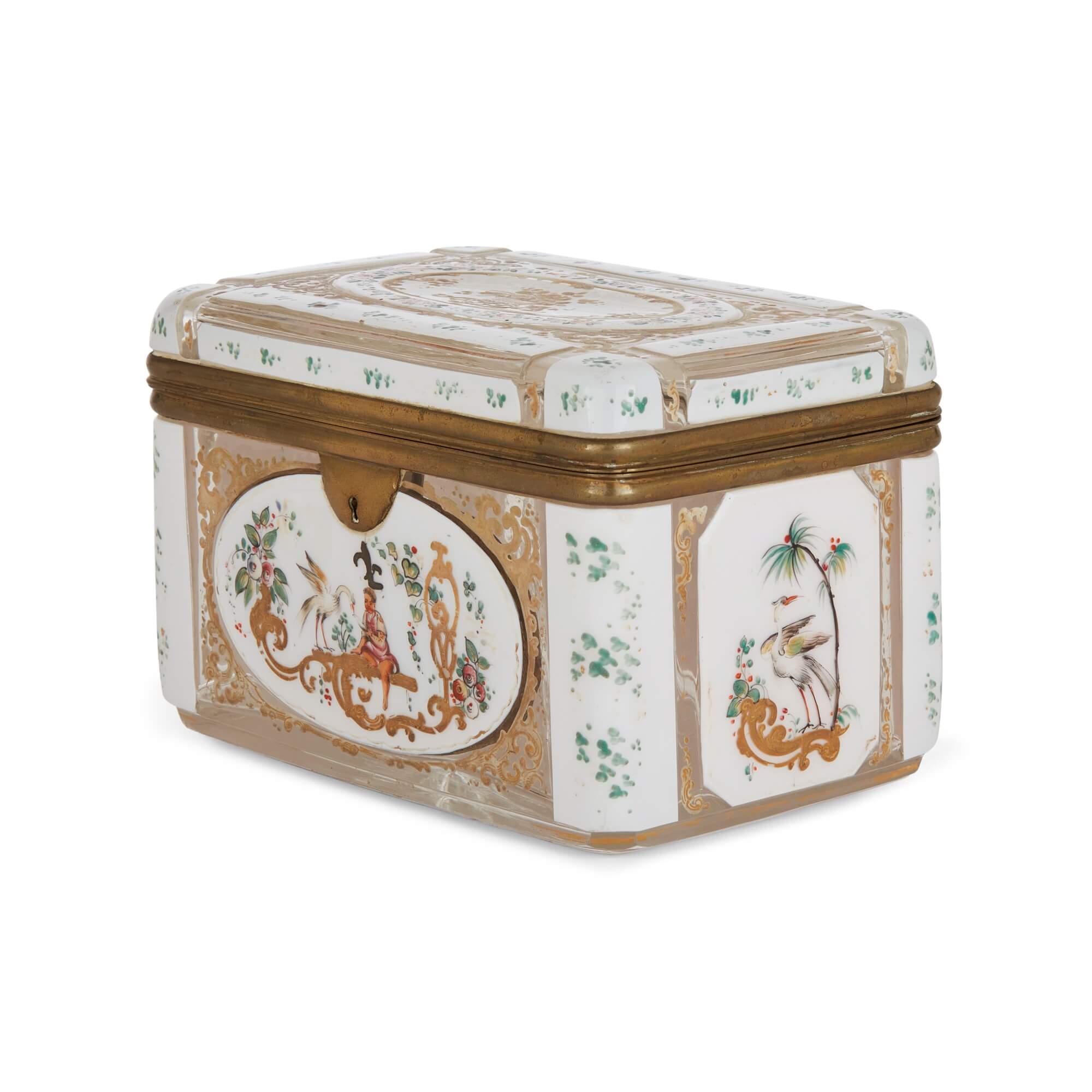This landscape-oriented color photograph captures a highly ornate, vintage tin or small chest, exuding historical charm. The rectangular container has rounded corners and features a hinged lid with dark brown trim lining both the top edge of the lid and the container itself. The box is crafted with elaborate detailing, including an ornate design on the top. A latch closure is prominently placed on the front. Positioned at an angle, the front corner faces the viewer, revealing an elliptical section with a gold and light green Asian-style motif on a white background. Both sides of the container display intricate artwork: the right side features a vertical octagonal shape showcasing a heron under a palm tree, characterized by its Asian aesthetic, while the left side depicts a crane next to a figure sitting on a wooden log. A recurring beige background with white trim adorns the panels, and green paint splashes are scattered on the corners, enhancing its antique allure. The overall photographic style is representational realism, and the background is virtually dropped, giving the impression that the box is floating against a white backdrop.